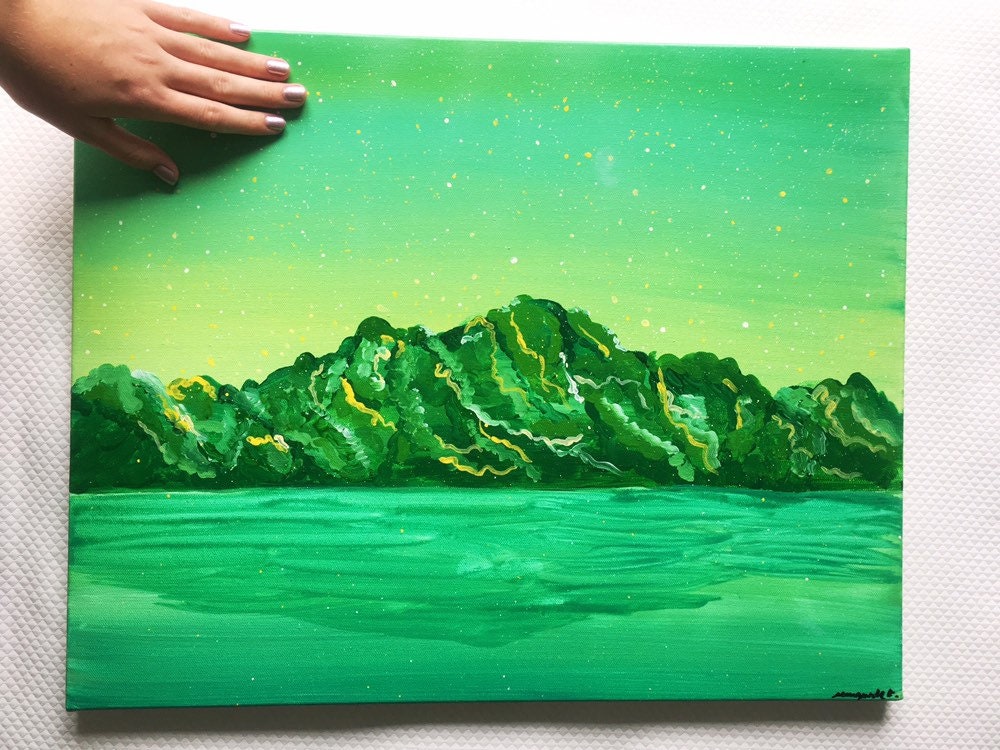In this horizontal rectangular image, a photograph captures a textured canvas painting being held up by a feminine hand with gold-colored fingernail polish in the upper left corner, pressing it against what appears to be a white, diamond-patterned fabric background. The painting itself is dominated by various shades of green, accented with hints of yellow and white. In the foreground, dark green waters reveal visible wave tops and reflections of the rocky cliffs above them. The mountainous landscape, drawn with darker green hues, features yellow lines along the ridges to add depth and detail. The sky transitions from a yellowish hue near the mountains to a darker green towards the top, speckled with white and yellow particles that evoke an ethereal atmosphere. A small black signature is visible in the bottom right corner of the canvas.